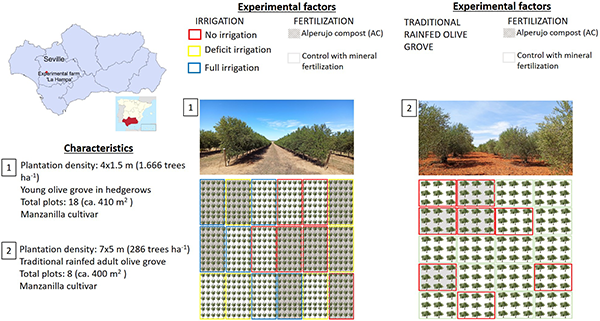The infographic displays experimental factors affecting olive groves in the Seville region of Spain. It features a small, light blue map of Seville in the top left corner, annotated with black text. Two plantation densities are described under "Characteristics": the first with a density of 4x1.5 meters (1,666 trees per hectare) for young olive and hedge groves, covering 18 plots; the second with a density of 7x5 meters for traditional rain-fed adult olive groves, covering 8 plots. Both use the Manzanilla cultivar. 

Central to the infographic are two contrasting photos of agricultural lands. The left image depicts a farmland with light brown soil and clearly defined tree rows, while the right image shows an area with orange soil, loosely defined rows, and some clouds in a blue sky. Below these images, tree layouts are sectioned off in red, blue, and yellow outlines, and filled with either gray or white, indicating different irrigation and fertilization treatments.

The legend at the top explains these experimental factors. For "Irrigation," a red outline indicates no irrigation, yellow denotes deficit irrigation, and blue signifies full irrigation. Under "Fertilization," gray fill represents Alperujo compost, and white fill indicates control with mineral fertilization. The right column further explains traditional rain-fed olive grove fertilization using the same gray and white color scheme.